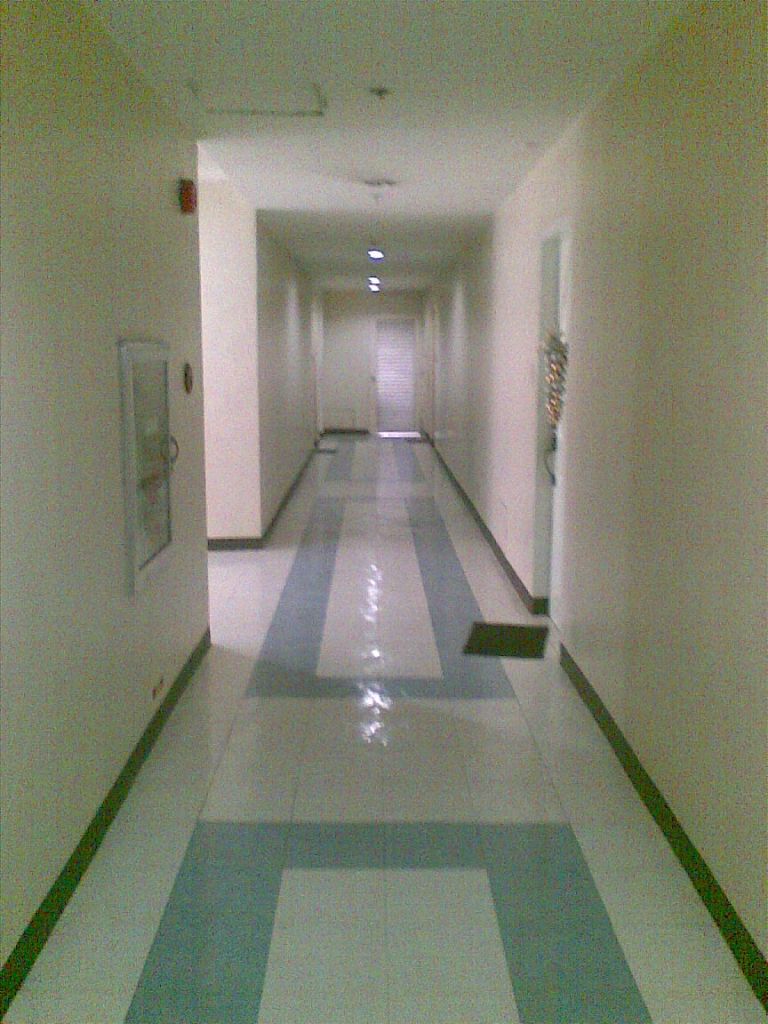This image depicts a long, narrow hallway that is likely part of a medical facility or an older apartment building. The hallway features white or off-white walls and a ceiling equipped with fire sprinklers and lights. The floor is adorned with a blue geometric square pattern repeated three times on a predominantly white tiled surface, bordered by a green baseboard. On the left-hand side of the hallway, there is an entryway, a fire alarm high on the wall, and a fire hose box with a handle, along with other unclear objects. The right-hand side of the hallway showcases a door adorned with a wreath and an askew doormat below it. At the far end of the hallway, there is another door. The hallway is clean but appears old and dated, with a somewhat dim lighting ambiance.